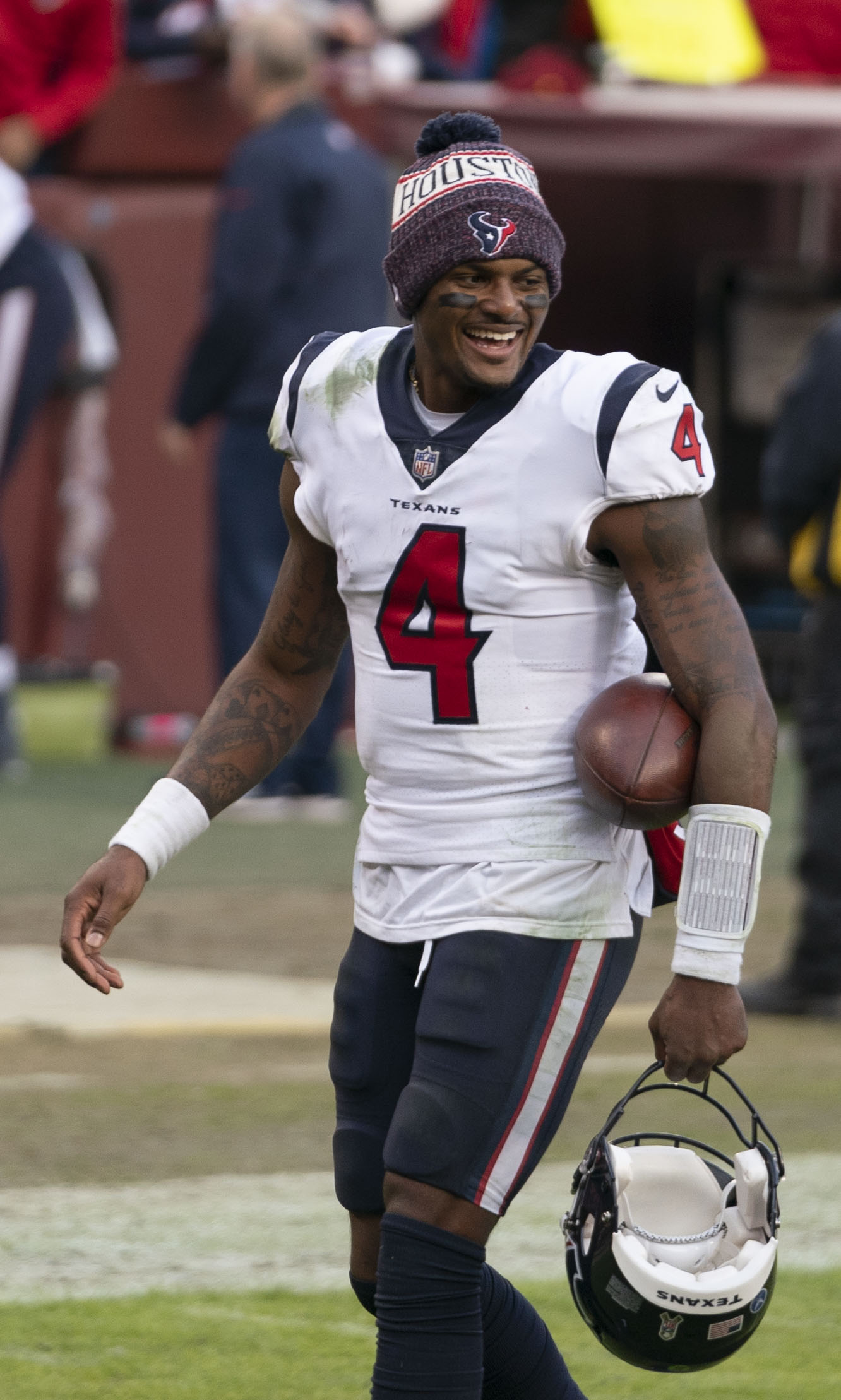In this vibrant photograph, a football player dons a white Houston Texans jersey with navy blue accents and the number 4 prominently displayed in red on his chest. The Nike swoosh and NFL logo adorn the shoulders and collar area of the jersey. The player, an African-American, is captured on a green football field with white markings, walking briskly while carrying a brown football securely between his waist and elbow. He is also holding a dark blue helmet emblazoned with the Texans logo in his other hand.

His uniform includes navy blue pants with red, white, and blue stripes running down the sides. Both his arms are adorned with tattoos, and he sports white wristbands. Black eye black is visible under each eye, and he wears a navy beanie with a white band reading "Houston" along with a small embroidered bull or steer symbol in front.

The background is blurred, showing a typical stadium scene with fans in the stands and individuals in the dugout or bench area. A man in a navy blue tracksuit and an older, balding coach with gray hair are slightly visible among the indistinct details. The player's demeanor is cheerful and relaxed, smiling and looking to the right, providing a sense of a candid moment during a break in the game.